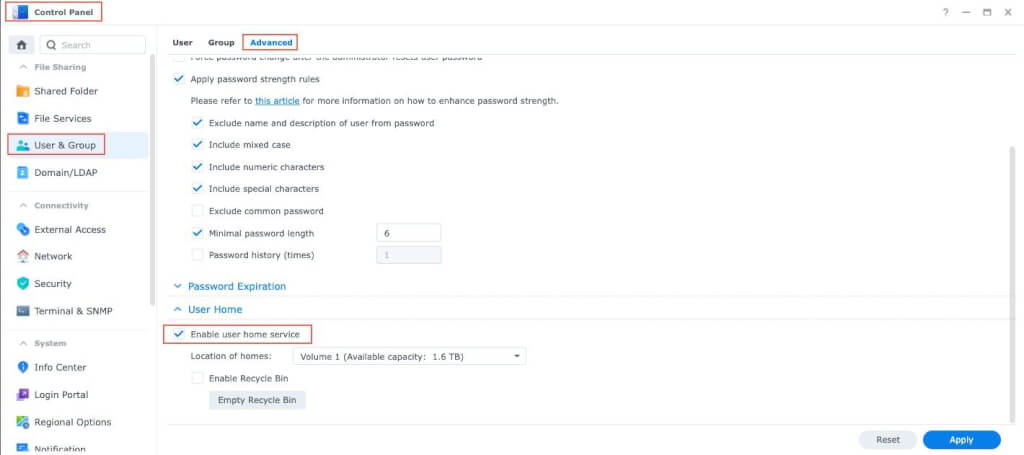**Caption:** 

This image appears to be of a detailed control panel interface, likely from a server management or network administration system, potentially Linux-based. The interface has a white background with a horizontal band of text on the left side. The top of the interface reads "Control Panel" and offers multiple options including "File Sharing," "Shared Folder," "File Services," "User and Group," which is highlighted in red, among many others such as "Domain," "External Access," "Network," "Security," "Terminal," and "Info Center."

To the right, the "User Group" section and the sub-option "Advanced" are highlighted. Below this, there is a list of security options with checkboxes. The options include:

- Apply password strength rules (ticked)
- Exclude name and description of user from password (ticked)
- Include mixed cases, numeric characters, and special characters (all ticked)
- Exclude common password (not ticked)
- Minimal password strength (ticked)
- Password history times (not ticked)
- Minimum password length set to six

Further down, "Password Expiration" is highlighted in blue. Another section called "User Home" outlines enabling user home service (ticked and highlighted in red), specifying its location as "Volume 1" with an available capacity of 1.6 terabytes. The option to enable the recycle bin is not ticked.

At the bottom of the interface, there is a gray "Reset" button with black writing and a blue "Apply" button with light gray writing. Besides these elements, there are control icons for closing and maximizing the window at the top. The intricate details suggest a comprehensive system configuration page.